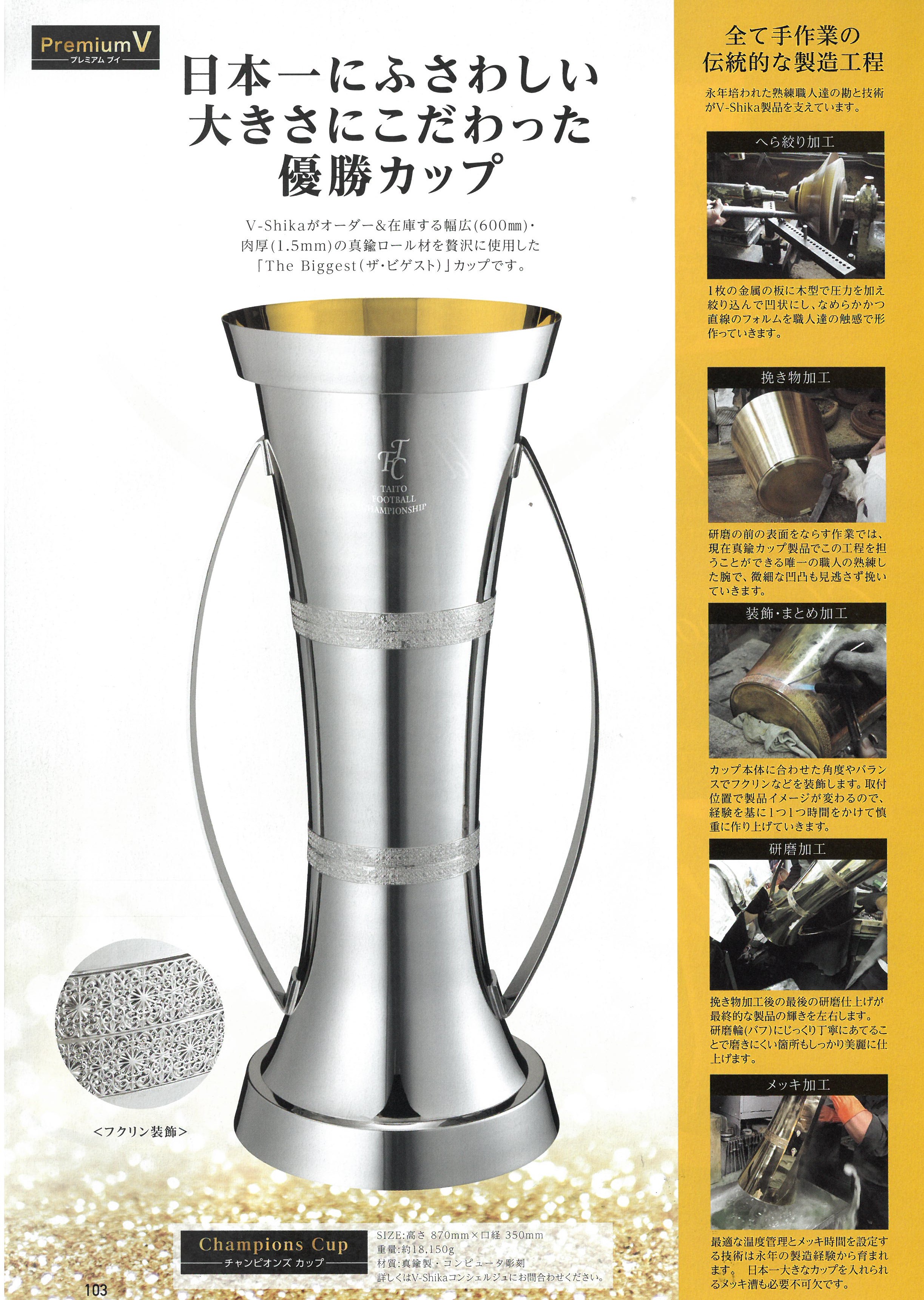This photograph, measuring approximately 4 by 7 or 8 inches, displays a tall, metallic trophy, possibly made of silver, with a cylindrical body that flares out at the end. The trophy features two handles, one on each side, and is intricately engraved with various details. At the top left of the image, "Premium 5" or "Premium V" is written in gold within a black rectangle, while at the bottom, the words "Champion's Cup" are displayed in a similar fashion. The main writing on the image consists of black characters in either Chinese or Japanese, suggesting that most of the text is in a language other than English. To the right of the central figure is a vertical orange bar containing five smaller square photos, each depicting different stages of the trophy's production process, from initial shaping on a lathe to the final polishing. A human hand is visible in the main photograph holding the trophy, adding a scale reference, and there is a possible indication of it being slide number 103 at the bottom. The background is predominantly white, highlighting the trophy's lustrous finish and detailed craftsmanship.